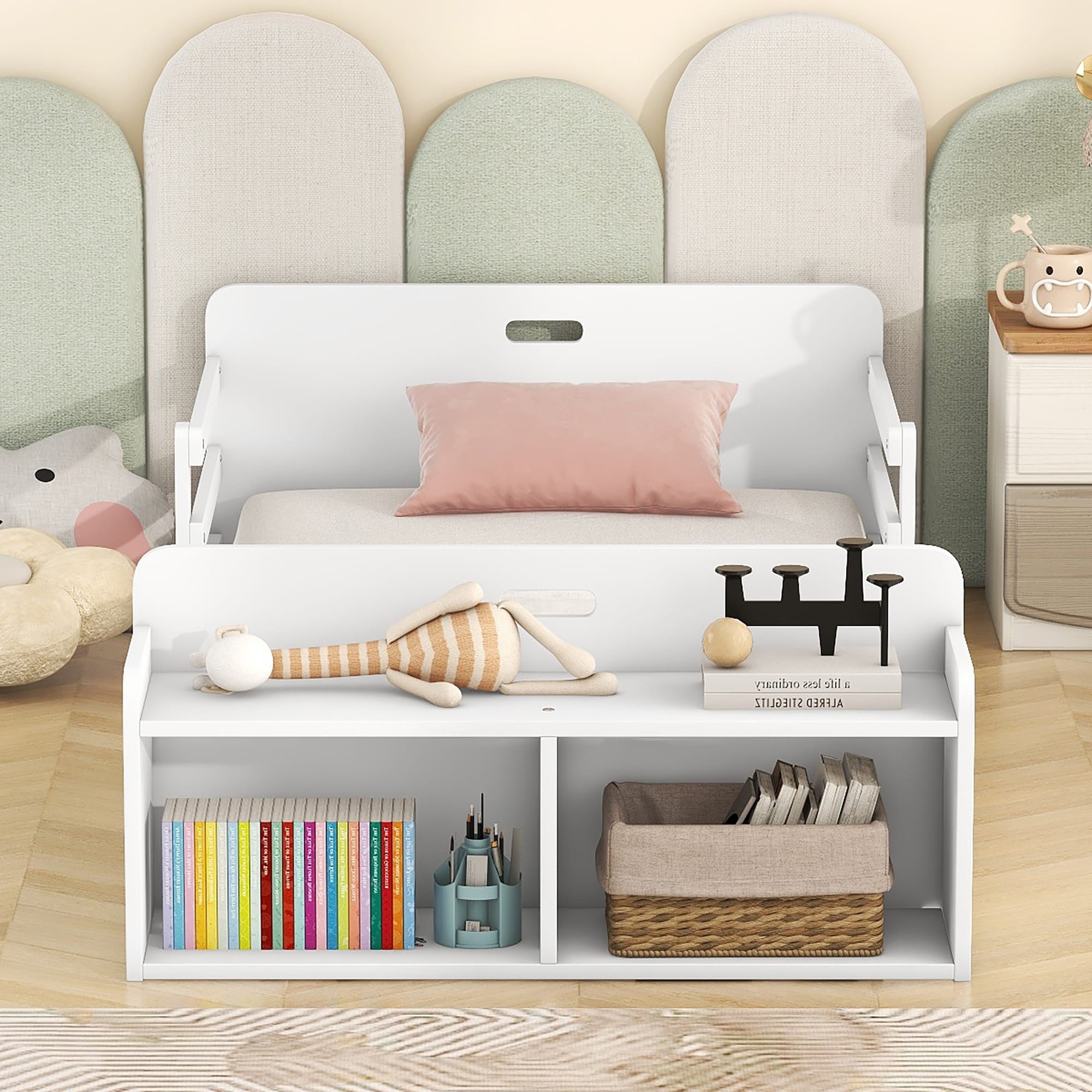The photo depicts a cozy and warmly decorated children's room with light wood flooring. The walls are painted a light yellow, and feature large scalloped pillars that alternate between pastel green and off-white, giving a playful, fenced appearance. In the center of the image, there's a small white bench with a beige seat cushion and a long pink throw pillow placed on it. In front of the bench is a white storage shelf that has two open cabinets at the bottom and a shelf on top, housing various items. Up against the wall, lined with patterned headstone-like decorations, is a cute white bed adorned with a sheet and a salmon-colored pillow. Next to the bed, there's a small nightstand with a tan, wide-mouthed mug featuring black eyes sitting atop it. At the foot of the bed, you spot a multi-colored throw rug, and on the left-hand side of the bench shelf, there's a collection of colorful books. On the bottom right, there’s a woodgrain book container and a stuffed animal figure, enhancing the whimsical and inviting atmosphere of the room.